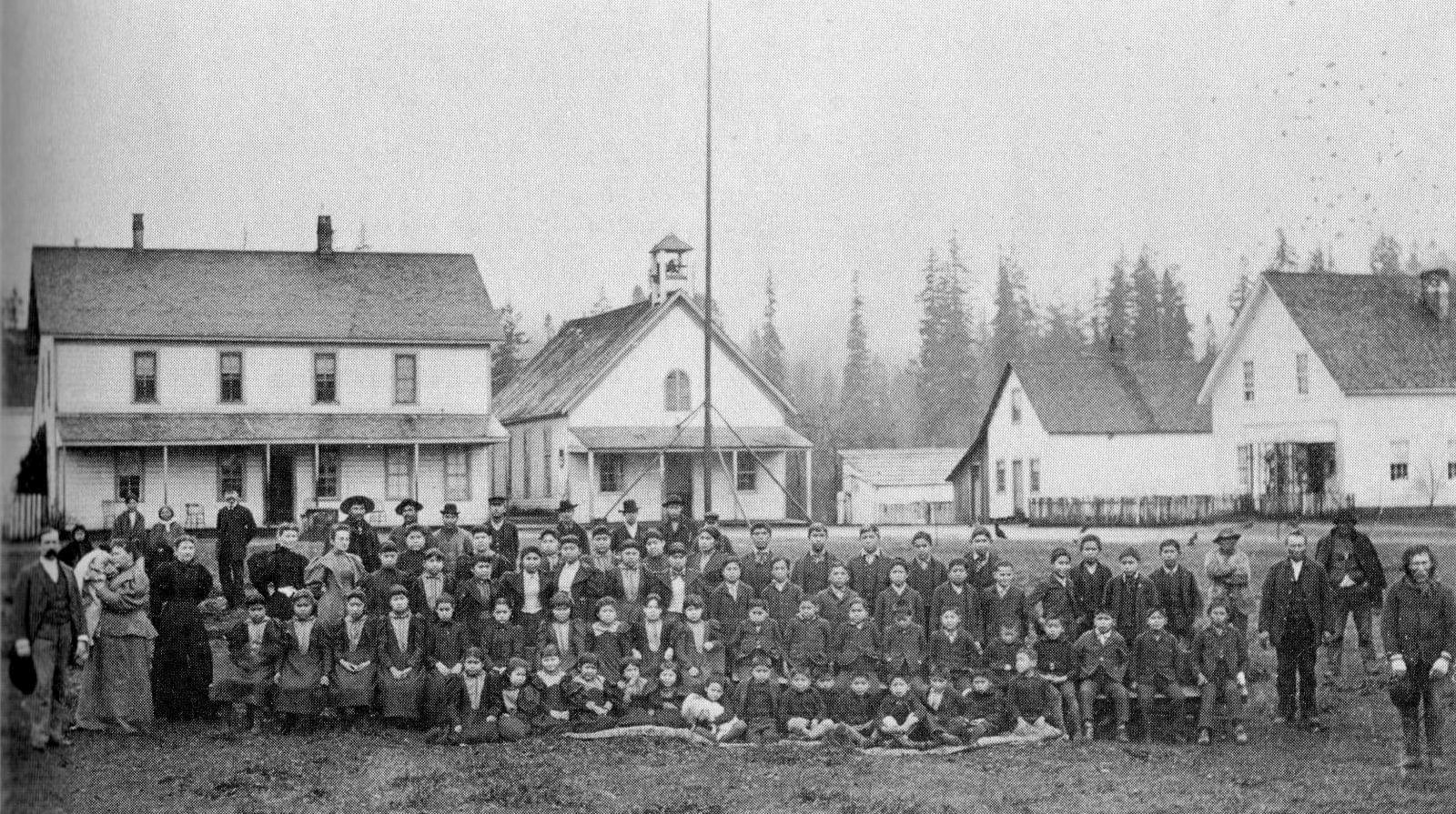This old black-and-white photograph captures a historical moment featuring a group of people, predominantly children, assembled in an outdoor, grassy area. In the foreground, there is a noticeable line down the center of the image which might be a pole or a crease from age. Clustered around this line are rows of children, with the front row sitting or kneeling on what appears to be dirt and grass. Behind these children, some adults are also seated, and further back, there are more adults standing. To the bottom left of the photo, three adults, both men, and women, are prominently standing. To the right of them, children are organized in four rows: the first row sitting or kneeling, the second row sitting, and the last two rows standing. To the far right, another small group of three adults is standing facing the camera.

The backdrop features a series of buildings. On the left, a large two-story building with windows on both floors and a central door takes up considerable space. Next, to the right, a smaller building with a steeple stands prominently. Farther right, there are two more white buildings positioned at an angle, revealing both their fronts and sides. Beyond these structures, a grove of pine trees is visible, rising above the rooftops and filling the gaps between the buildings, with a gray sky overhead. The composition and organization of people and buildings suggest a formal gathering, possibly for a group photo, capturing a significant moment in time.